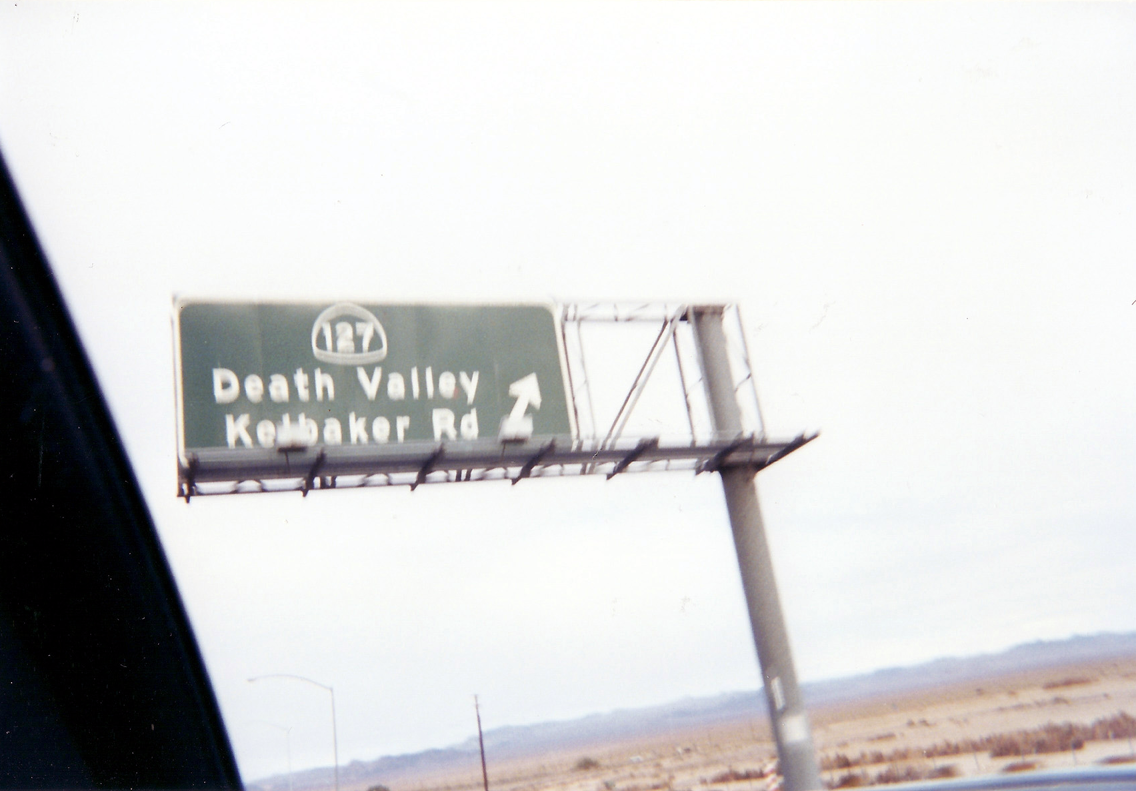This grainy daytime photograph, taken from the perspective of a vehicle traveling on a highway, prominently features a large green sign mounted atop a towering metal pole. The sign, in white font, reads: "127 Death Valley, Kelbaker Road" with an upward-pointing arrow. The backdrop showcases a barren desert landscape characterized by patches of brown grass and scattered sand. A light pole and what appears to be a power pole are faintly visible in the distance. At the base of the metal pole holding the sign is a small white object. The horizon is framed by a rugged, mountainous terrain. Despite the image's graininess and slight blur, the essential details of the desolate yet striking scenery are discernible.